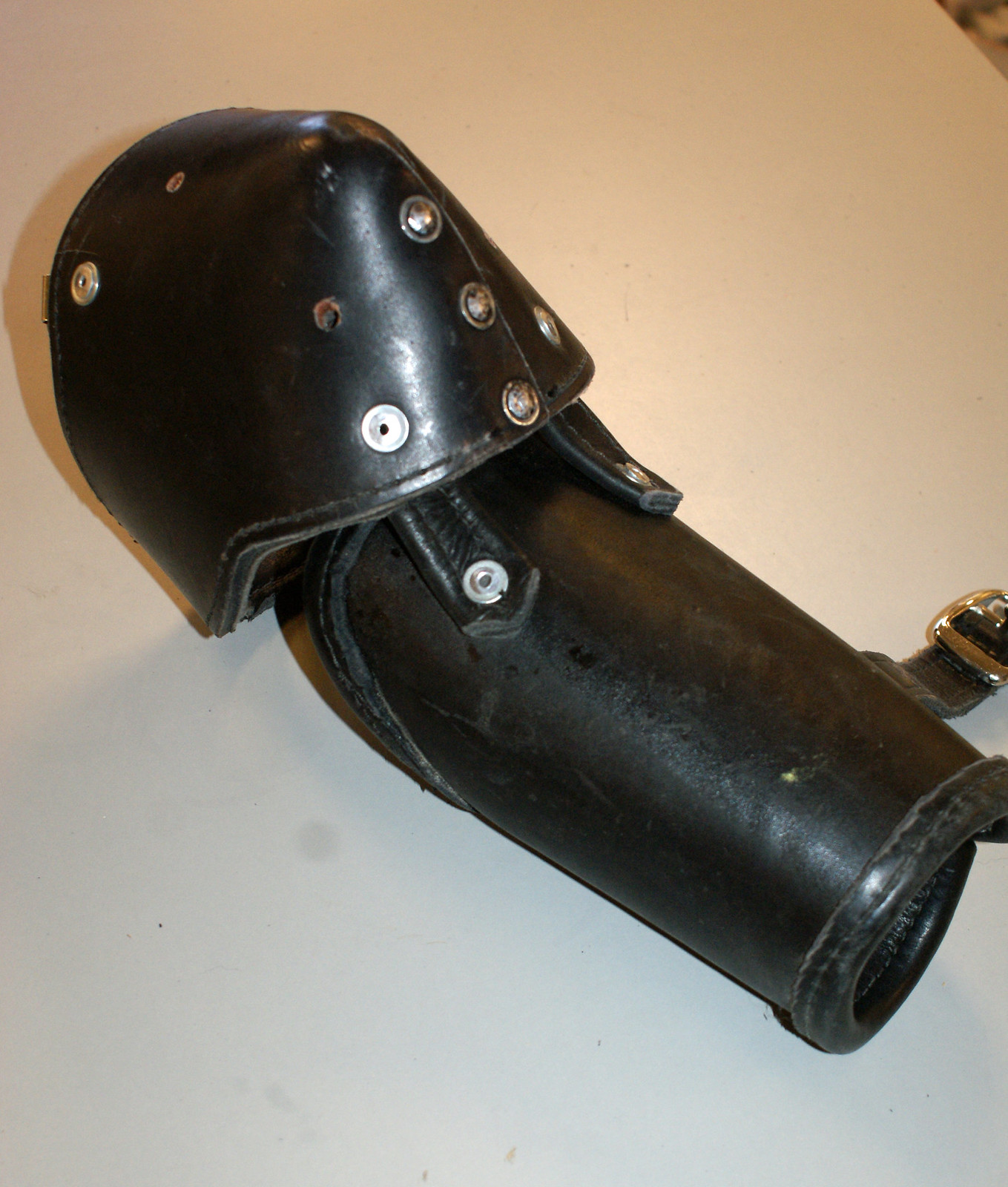The image shows a close-up of a detailed piece of black leather body armor, centered and angled from the upper left to the bottom right on a white background. The armor appears to be a combination of different parts: one section looks like it could fit over the shoulder, while another cylindrical piece seems designed for the bicep or leg, likely functioning as a knee pad with an attached shin guard. The black leather construction is accentuated with numerous silver metal rivets, some of which appear to be missing. Additionally, there are buckles visible at the base of the armor, suggesting it can be strapped securely around the body. At the front, there's a distinctive component made of rolled-up red leather, integrated into the design, which adds a unique visual element to the otherwise predominantly black piece.